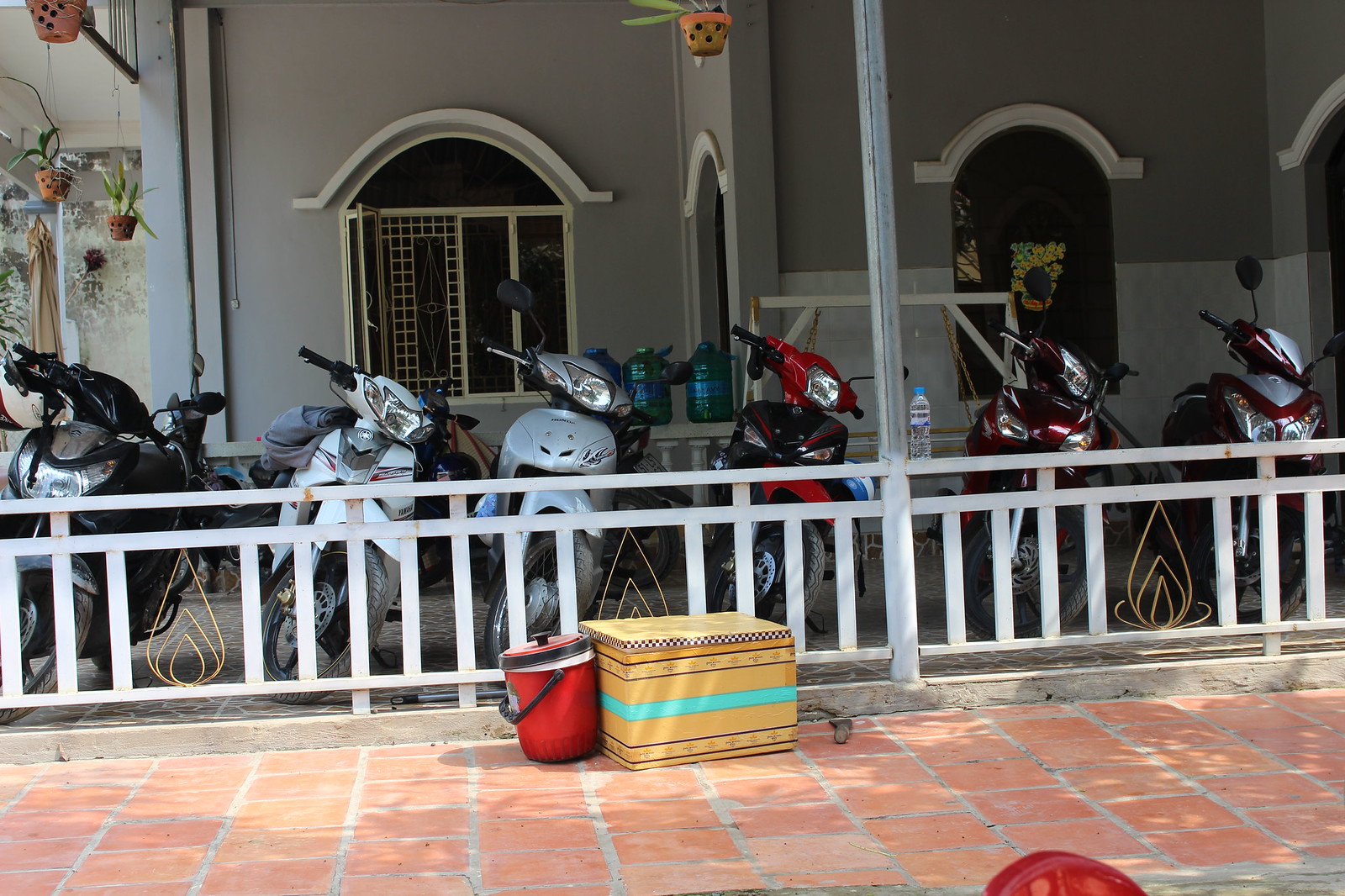The image captures an outdoor scene featuring six motorcycles parked in a row against a white fence with yellow teardrop decals. The motorcycles vary in color: a black one on the far left, followed by white, silver, bright red, and two maroon ones. A gray building with arched windows framed in white forms the backdrop. The windows have white trims and rest above darker white windowsills. Below the motorcycles, a brick patio extends across the scene. In the center of the patio, prominently positioned, are a yellow box with a teal stripe and a red cylindrical container with a black handle. Potted plants in brown terracotta holders dangle from an unseen overhead structure, adding a touch of greenery to the setting.